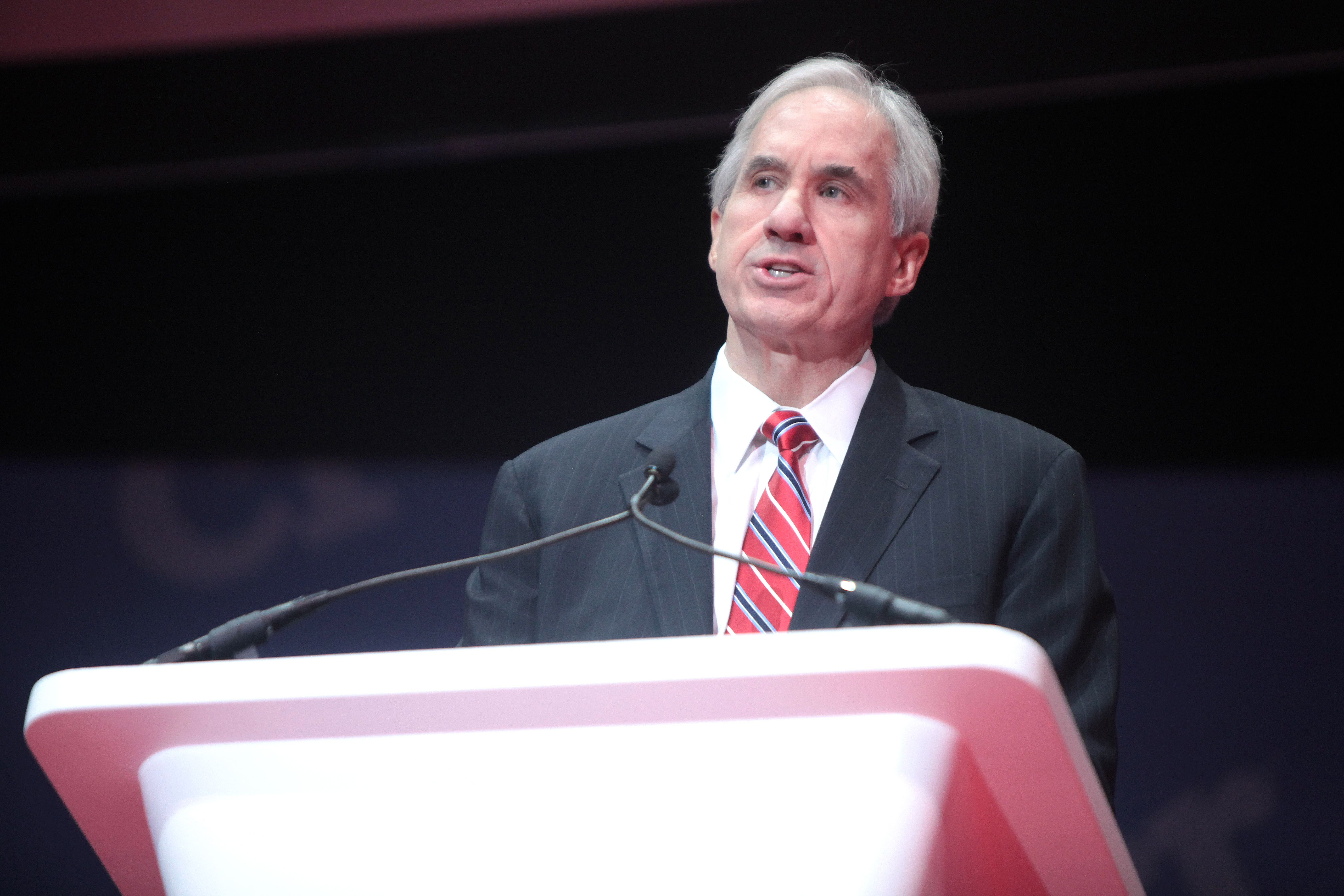An elderly man, likely in his 60s or 70s, stands behind a white podium with two long, slender microphones angled towards him. He has silver hair, thick dark bushy eyebrows, and appears to be speaking. He is dressed in a white collared shirt, a red tie with blue and white stripes, and a dark black jacket. The background of the image is primarily black but faded, making the text indistinguishable. The podium is centrally placed, extending slightly more to the left, and the setting suggests a formal speaking event.